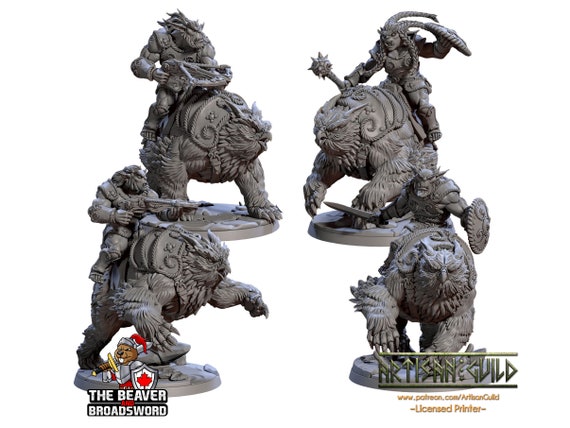This product photograph showcases four meticulously detailed grey miniatures, designed for tabletop gaming, such as Dungeons and Dragons. The figures appear to be either clay-crafted or 3D printed, awaiting a personal touch of paint. Displayed against a solid white background and surface, the miniatures appear to float in a seamless void.

Each of the four miniatures depicts a goblin-like creature wielding weapons such as shields, crossbows, and swords, mounted atop a creature resembling a bear with an owl’s face, reminiscent of an owlbear. This striking ensemble is perfect for game enthusiasts looking to add unique pieces to their collection.

The photograph includes a logo in the bottom left corner featuring a knightly cartoon beaver holding a sword and shield, detailed with a red maple leaf, symbolic of Canada, alongside white text that reads, "The Beaver Broadsword." In the bottom right corner, there's gold text reading "Artisans Guild," followed by a URL "www.patreon.com/Arthanguild," noted in a runic font.